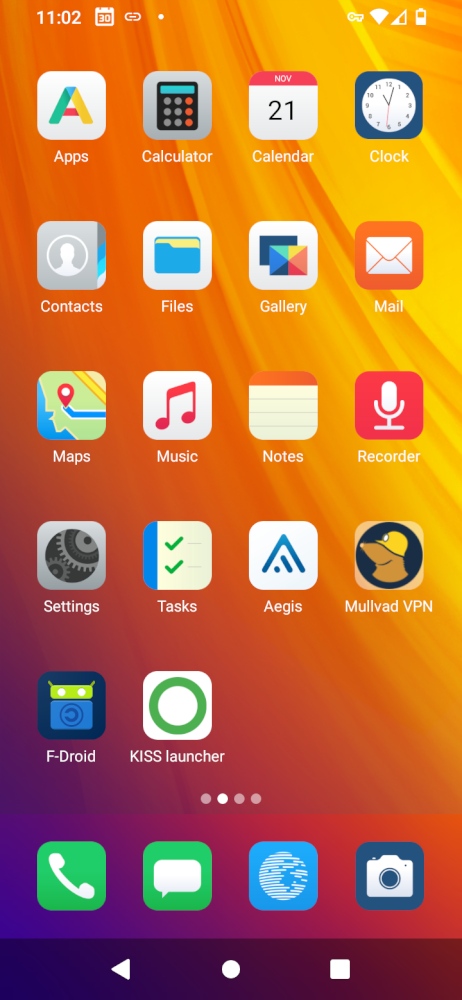The image shows a detailed screenshot of a smartphone's home screen, set against a vibrant ombre background that transitions from deep purple in the bottom left corner to reds and lighter reds, culminating in a yellowish-orange hue in the top right corner. The screen displays the time as "11:02" and features a small calendar icon showing the date "30". In the top right corner, there are status icons including a key (likely indicating a password manager or security app), a Wi-Fi signal, cellular signal bars, and a battery indicator. 

The app icons on the screen are neatly organized and include: an "A" for apps, Calculator, Calendar, Clock, Contacts, Files, Gallery, Mail, Maps, Music, Notes, Recorder, Settings, Tracks, Tasks, Aegis (spelled A-E-G-I-S), Malbad VPN, F-Droid, and KISS Launcher. Additionally, there are icons for telephone, messaging, web browser, and camera. At the bottom row of the screen, navigation icons for back, home, and recent apps are displayed in the form of a back arrow, a white circle, and a square, respectively.